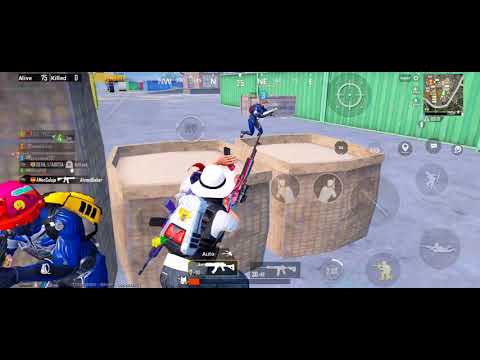A video game screenshot features a third-person shooter scene reminiscent of Fortnite. The main character, designed with a white hat and white backpack possibly doubling as a jetpack, is positioned behind wooden crates. This character wears blue jeans and holds several guns at their side. Across from them, separated by two large square barrels, is another character decked out in a blue outfit, a yellow backpack, and a pink helmet adorned with an emoji. The backdrop includes lime green storage containers, with additional blue, red, and white ones visible in the distance. The ground is gray, resembling pavement, and the user interface displays multiple guns, a radar, a map in the upper right corner, and various scores and indicators. White text naming players can also be seen on the left side of the screen.